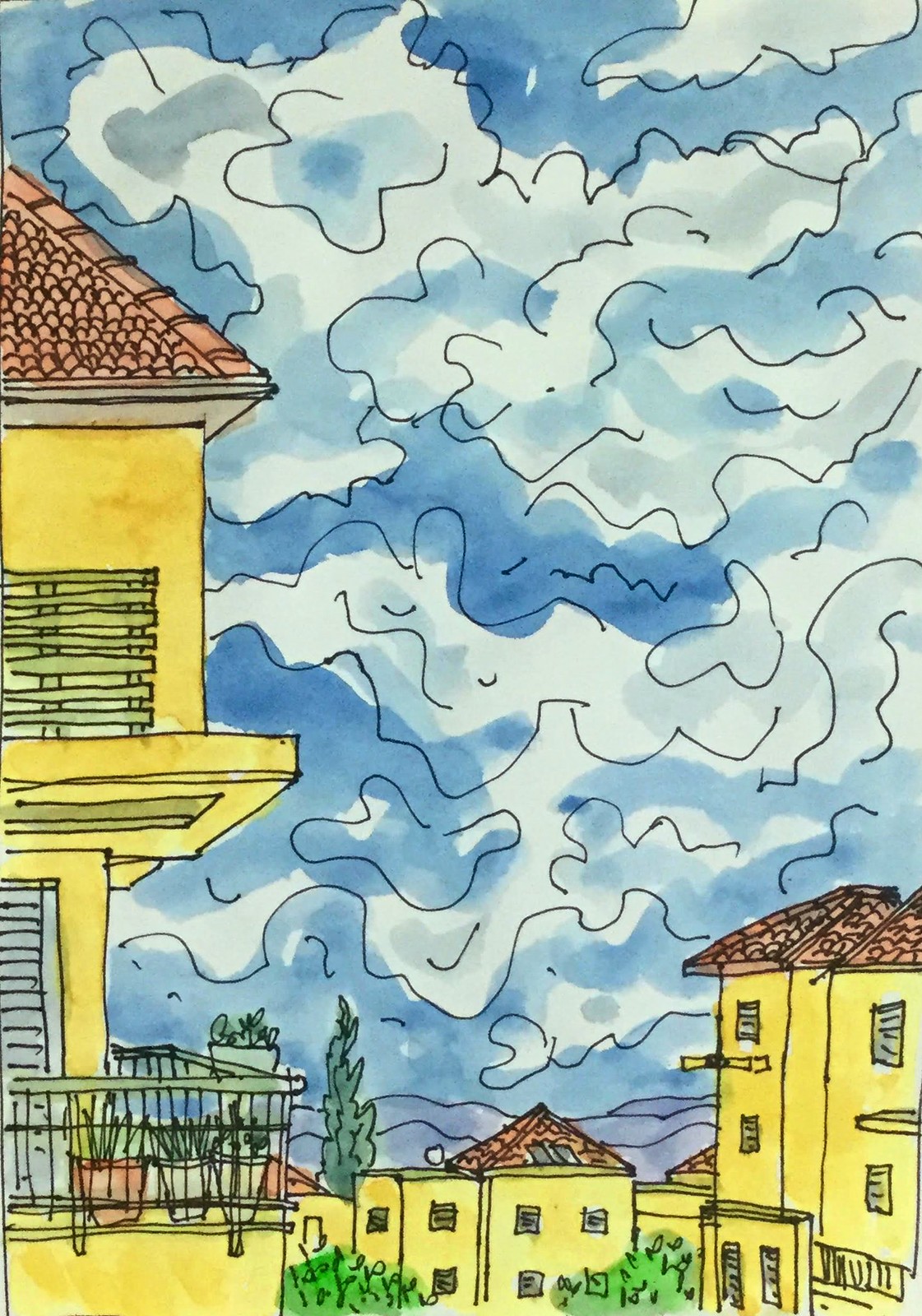This is a detailed drawing of an old-time city or town in a portrait orientation. The image features several yellow dwellings with orange-red, clay-tile roofs. At the bottom and on the left, right, and center of the image, there are multiple buildings, including at least one two-story structure with two rows of square windows. One prominent building, closer to the viewer, includes a balcony with four potted plants and Spanish-style railings. The sky above the dwellings is an array of blue hues, both dark and light, with clouds outlined in black and filled with white and light blue. Greenery appears at the bottom of the image, possibly indicating the tops of trees or bushes flanking the middle section of the artwork. The piece seems to be created with ink and colored with paint.